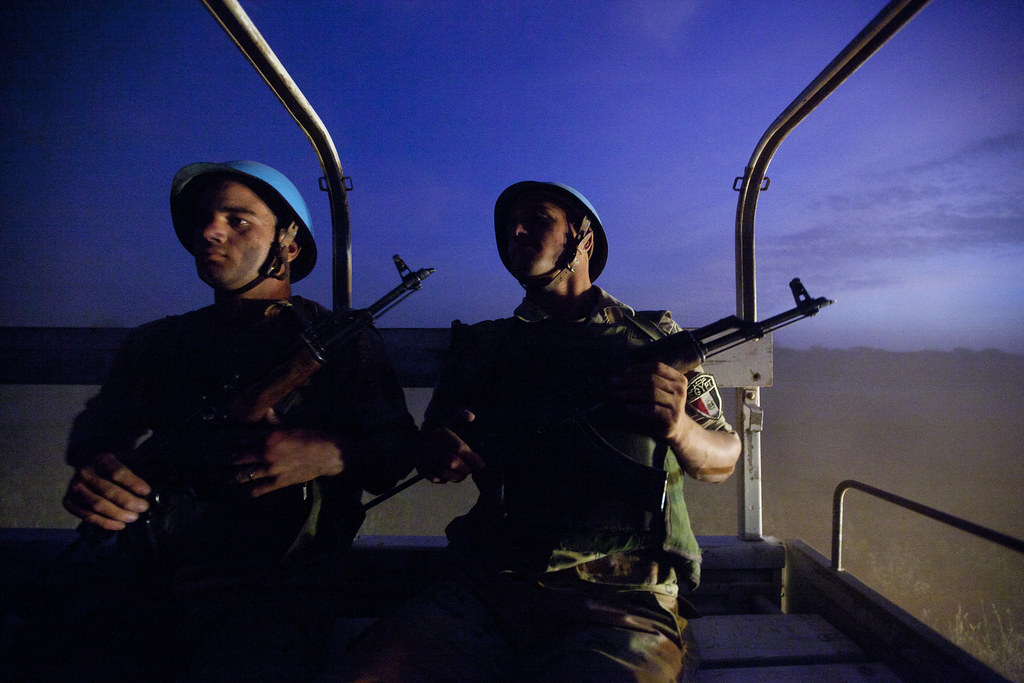This is a detailed color photograph depicting two soldiers in army-issue uniforms, situated on what appears to be a boat on a river at dusk. The sky above them transforms from deep blue to purple, indicating that the sun has recently set. Both men are adorned with light blue helmets secured with chin straps and are holding guns pointing across their chests while they look in the opposite direction.

The soldier on the left, partially obscured by dim lighting, has his hands on a backpack in front of him from which his gun protrudes. The soldier to his right grips his weapon directly. Both are seated on what appears to be a vehicle, suggested by the visible wooden railing along the edge. The murky water in the background adds to the sense of a twilight patrol. A patch on one soldier's arm reads "Egypt," hinting at their possible identity as Egyptian soldiers on duty. The atmospheric tones of the photograph, ranging from dark shadows to the faint light on the horizon, complement the mysterious and vigilant posture of the men.